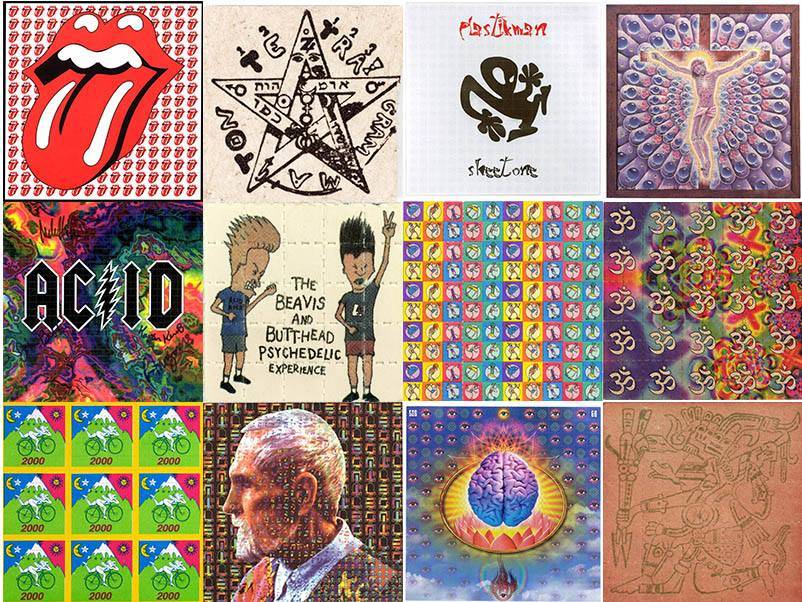The image displays a meticulously arranged collage of twelve square-shaped, color illustrations, laid out in a 4x3 grid within a landscape orientation. In the top left corner, the iconic red lips and tongue logo of the Rolling Stones stands out prominently. Moving to the right, the next illustration features a star accompanied by some foreign or cryptic text, possibly reading "Tetra Graham." Next in line, there is a depiction of a black alien figure with the words "Plastic Men" above it and “Street to Me” below. The top right corner is occupied by a vivid image of Christ on the cross, surrounded by multiple eyes, likely referencing the band Tool. 

Continuing down, the second row begins with an illustration displaying the text "ACID" with a lightning bolt in psychedelic colors. Adjacent to it is a comically surreal depiction titled “The Beavis and Butthead Psychedelic Experience." The next square illustrates a colorful array of small, green, pink, and yellow squares interspersed with tiny human figures. Completing this row is an image featuring the number "30" repeatedly in various colors.

The bottom row starts with an homage to Albert Hoffman’s discovery of LSD, titled "Bicycle Day," featuring bicycles and the year 2000. Next to it is a profile view of a man, followed by a vibrant visualization of a brain. The final image in the collage is a dynamic depiction of a man with multiple arms, symbolizing a sense of fragmented motion. 

Taken together, the collection of these iconic and psychedelic artworks suggests a diverse array of cultural references, possibly related to blotter paper used for LSD, and features a mix of rock band logos, abstract art, and pop culture icons.